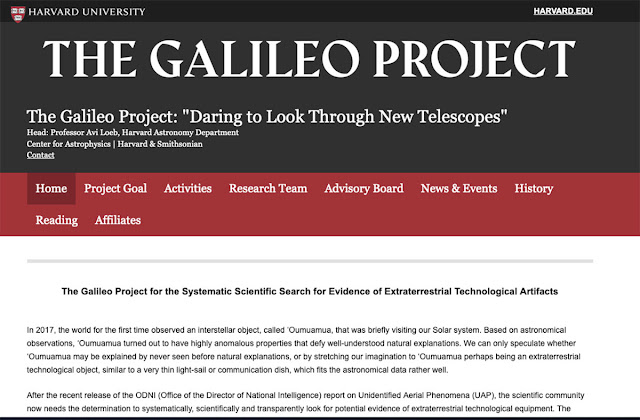In this captivating image, a post from Harvard University proudly showcases the headline "The Galileo Project." The text beneath sets the stage for an exciting journey into astronomical exploration: "The Galileo Project, daring to look through new telescopes." This initiative is spearheaded by the Harvard Astronomy Department, in collaboration with the Center for Astrophysics, Harvard & Smithsonian.

The image outlines several key navigation links including Contacts, Links, Home, Project Goal, Activities, Research Team, Advisory Board, News & Events, History, and Reading. Collectively, these resources provide comprehensive insights into the project's multifaceted approach.

The core mission of The Galileo Project is explicitly stated: "The Galileo Project for the Systematic Scientific Search for Evidence of Extraterrestrial Technological Artifacts." 

A historical note adds grandeur to the announcement by referencing a groundbreaking astronomical event from 2017. For the first time, humanity observed an interstellar object named Oumuamua, which briefly visited our solar system. Astronomical observations revealed that Oumuamua exhibited highly anomalous properties, defying well-understood natural expectations. This mysterious visitor from another star system has motivated the scientific community to embark on this ambitious quest for extraterrestrial artifacts, with Harvard University at the forefront of this thrilling exploration.